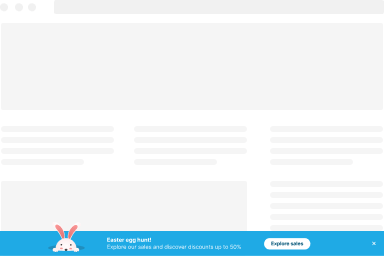This image appears to be a screenshot from a website experiencing technical difficulties, as it lacks typical elements such as icons, text, headers, and banners. The top left features three gray circles arranged horizontally, which likely represent icons. To their right is an empty gray bar. Below this bar is a larger rectangular gray box, also unpopulated. The main content area beneath these elements has a white background sprinkled with several small, empty gray boxes that suggest missing lines of text. In the bottom left corner, there is another empty gray box. Adjacent to this are more thin, gray lines that seem to indicate additional missing text. At the very bottom of the page, a blue bar contains text that reads "Easter egg hunt" beside an image of a white rabbit. The bar also has an 'Explore' button and an 'X' closeout button on the right side.